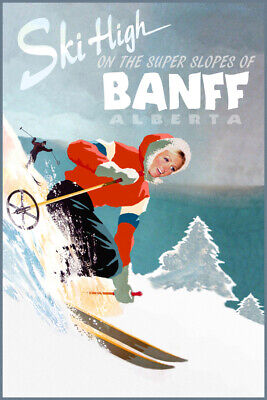This image is a vintage-style promotional poster for Banff, Alberta, featuring an animated woman skiing down a snowy mountainside. The skier, a white blonde woman, is dressed in a red coat with a fur-lined hood framing her face, and the coat's upper arms have distinctive white and blue stripes. She wears black pants, white gloves, and holds yellow ski poles. Her yellow and white skis kick up snow as she glides forward. In the background, a steep snowy hill extends out of view, with another skier, a silhouetted figure, descending behind her. The backdrop includes a blue sky, dark bluish mountains, and scattered snow-covered trees. Above the skier, in large white letters, the poster reads, “Ski High on the Super Slopes of Banff, Alberta,” emphasizing the thrilling ski experience offered in this Canadian province.